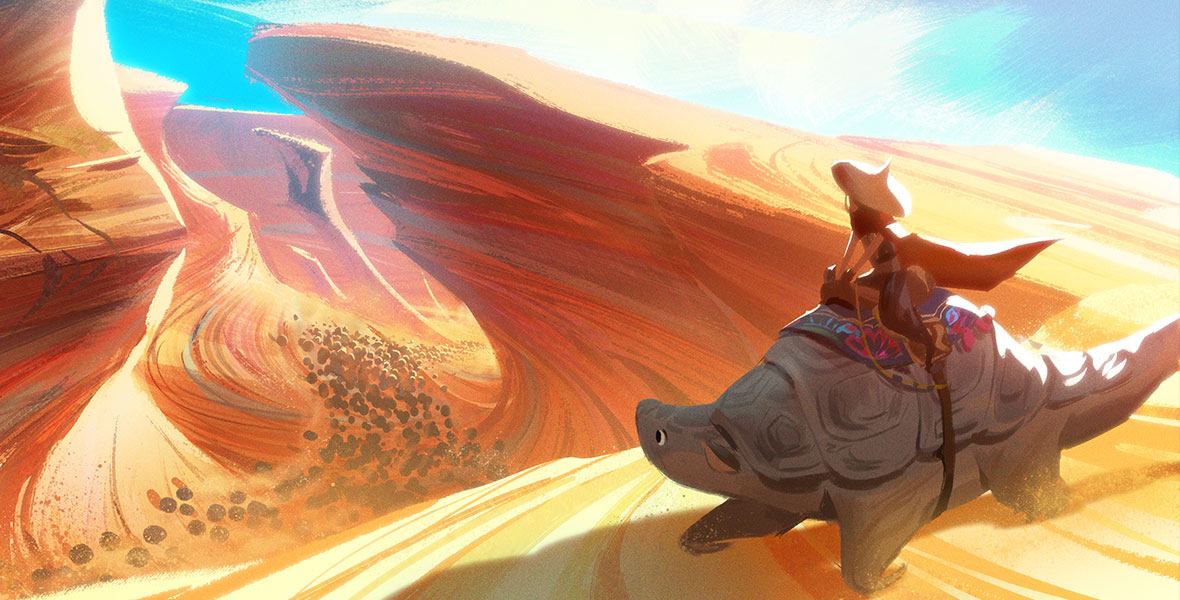This highly detailed animated drawing captures a scene set in the daytime desert, featuring a person of undetermined sex who might have a feminine appearance due to a midriff-baring brown shirt, coupled with brown pants and a striking red cape. The person also dons an Asian-styled conical hat, protective against the sun yet pointed in the middle, and has black hair. Seated on a brown saddle with a red and blue blanket underneath, the person rides a fantastical creature resembling a giant turtle or armadillo with a long tail, gray in color. The creature, showcasing black eyebrows and eyes, gazes upwards towards the sky alongside its rider. They are positioned atop a cliff overlooking a vast, windswept desert valley. Swirling rocky cliffs frame the background, extending down to the valley floor where numerous black dots, possibly herds of creatures, are scattered. The sky overhead is a clear blue, dotted with white clouds, adding to the wild and untamed essence of this expansive desert scape.